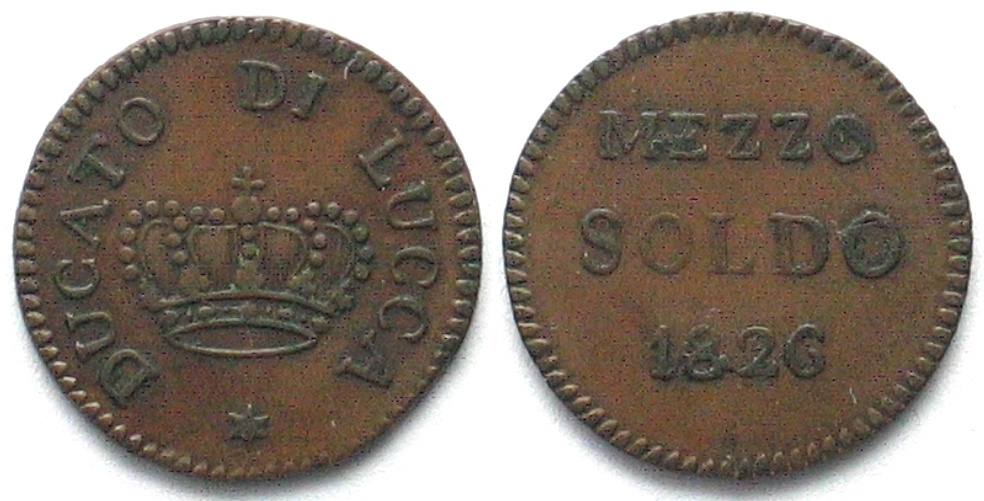The photograph, presented in landscape mode against a white background, showcases the two sides of a weathered, dark copper coin from 1826. On the left side of the image, the coin is inscribed with the words "Ducato di Lucca" encircling the edge, featuring an ornate king’s crown at its center and a six-pointed star situated at the bottom. The coin's edge is detailed with a triangle notch design. The right side of the image displays the reverse of the coin, where the text "Mezzo Soldo" is aligned in three descending lines, followed by the year "1826". The coins exhibit a considerable amount of rust and patina, highlighting their age and historical significance.